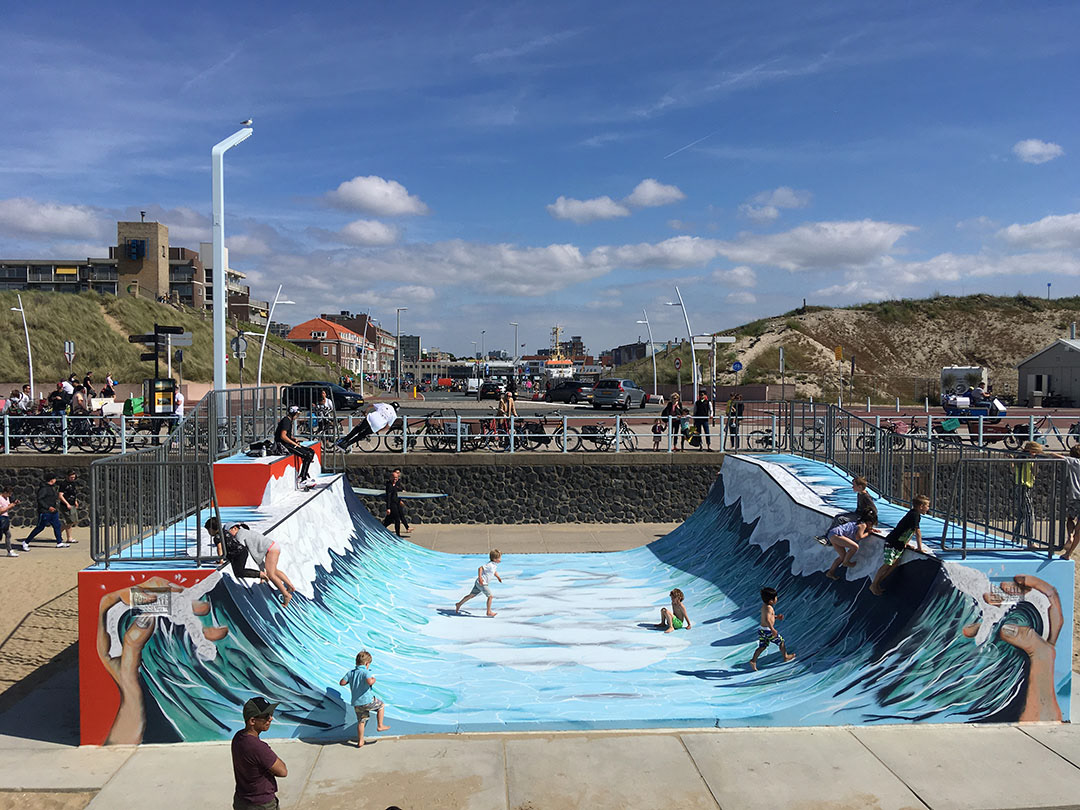The outdoor image showcases a vibrant and bustling skate park adorned with artistically painted waves, making the surface appear like an ocean being held by giant hands. The sky above is a medium blue with wispy and puffy clouds, setting a serene backdrop. On the left side, a taller, multi-story building that likely serves as a hotel dominates the hillside, while a series of buildings below suggests a mix of hotels and shops. In front of these structures lies a parking lot filled with various cars. The opposite hill, lower in height and covered with grass and dirt, is devoid of buildings but features a stone wall topped with a two-layered white fence where bikes are parked.

Central to the scene, concrete sidewalks frame the skate park, which doubles as an unusual and interactive art exhibit. This exhibit is actively explored by barefoot children running up and down the ramp, which is designed to mimic ocean waves. A seating area marked with blocks of red and white is situated on the left, while the right is bordered by a simple fence. People of all ages are seen engaging with the exhibit, some climbing, some perhaps skating, and others simply observing. The vibrant colors—from the blues of the sky and painted waves to the varied attire of the visitors—enhance the lively and communal atmosphere of this picturesque town setting.